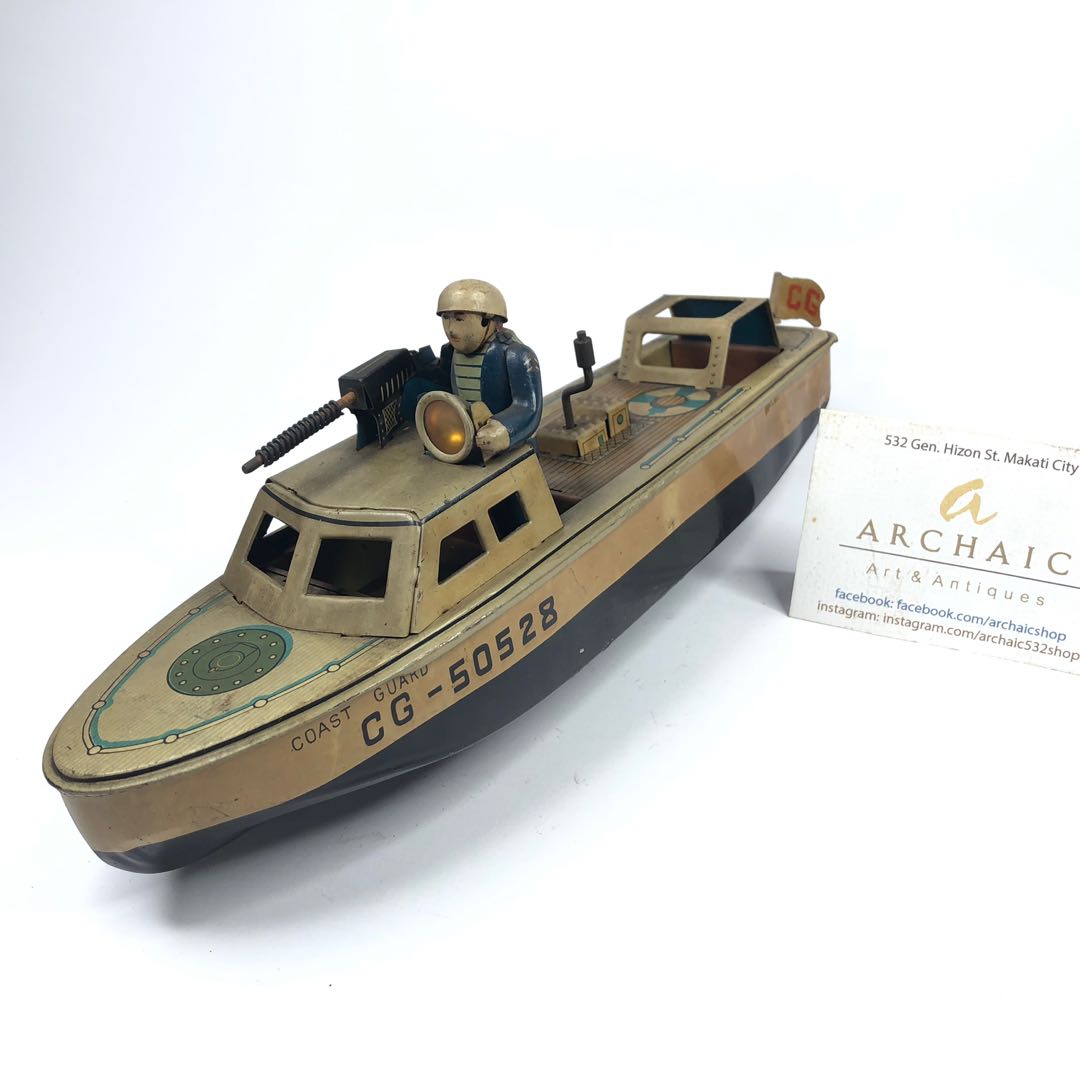This is an image of an antique toy model of a wooden Coast Guard boat labeled with "CG 50 528" on its side. The boat has a dark blue hull with an off-white, slightly weathered top, indicative of its age, possibly dating back to the World War II era. A detailed plastic soldier is depicted driving the boat, wearing a brown helmet and a blue jacket, and operating a machine gun and a yellow searchlight. The boat model also features a green hatch at the front and a flag with red "CG" text at the back, though the rear part of the boat is not visible in the image. The entire scene is set against a white background, and to the right of the boat is a business card from "Archaic Art and Antiques," indicating the piece is a collectible item. The business card includes contact details such as Facebook and Instagram information, linked to their shop "Archaic 532."